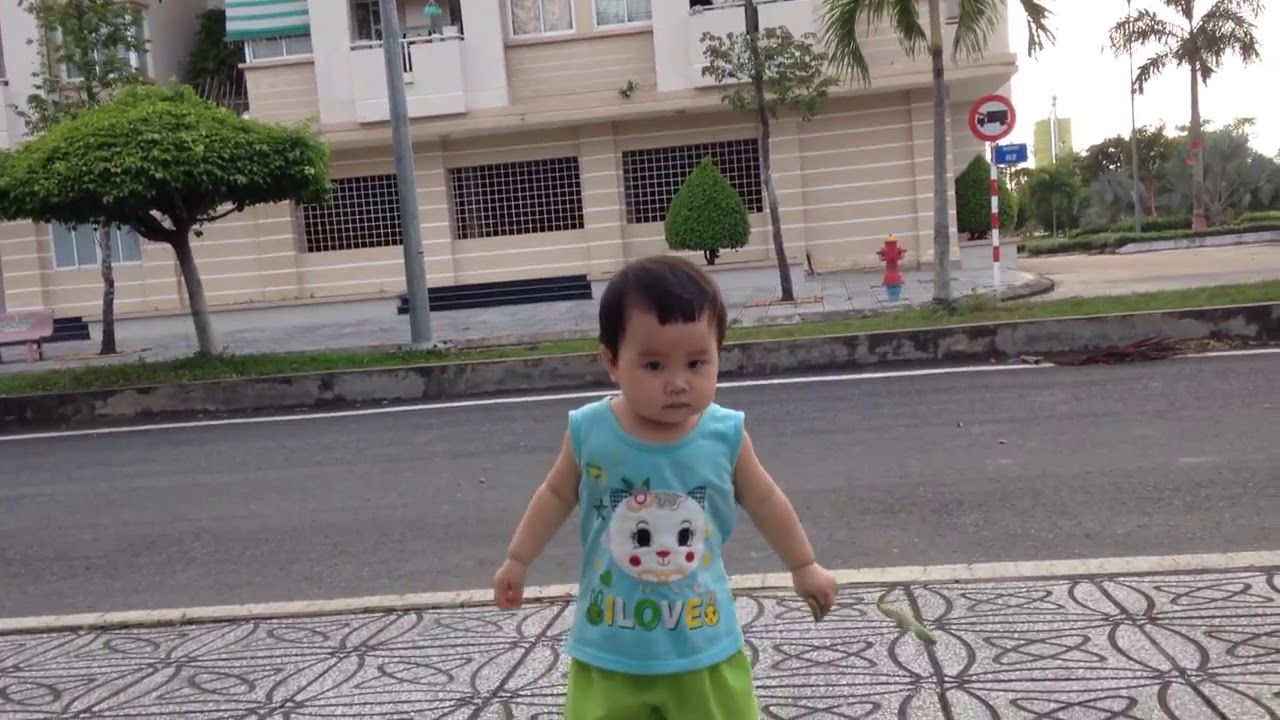This outdoor image captures a small child with short dark hair, standing on a decorative sidewalk that features various etched designs. The child, of either Asian or Mexican heritage, is wearing a blue sleeveless shirt adorned with two kittens flanking the words "I love" and green shorts. The child is looking directly into the camera. Behind the child, the neatly maintained sidewalk extends into a clean road, with a cement berm edging it. Further back, a stone wall, patches of grass, and a variety of trees can be seen, leading up to a taupe and white apartment building. Among the trees, there is a prominent power or lighting pole, signage including a "no truck" sign, and a fire hydrant near the building. The picture, slightly skewed counterclockwise, also offers glimpses of windows, balconies, and a partially visible sky.